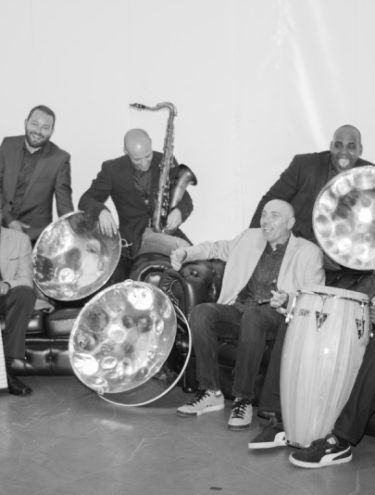The black-and-white photograph features a lively group of musicians, captured off-stage. The setting includes two couches, though only parts of them are visible due to the zoom. The scene is bustling with musical instruments and joyful expressions. 

On the left side, a partial view shows someone's leg, foot, blazer, and hand, hinting at a larger group presence. Behind this figure, a bearded man in a dark suit stands, smiling warmly. Beside him is a bald man, seated on the couch's armrest, holding a saxophone. He is dressed in a dark shirt, his arm resting on what appears to be a drum.

Across on the other couch, another bald man in a dark-colored suit stands, mouth open in an expressive smile, perhaps talking or laughing. In front of him, a man in a light-colored blazer, dark pants, and matching shoes sits engaged in conversation, his mouth open. Near him, a drum is placed beside someone's legs clad in Puma sneakers, though the rest of this person's body is not visible.

The background consists of a dark gray floor and a plain white wall, keeping the focus on the musicians. Throughout the image, various instruments including steel drums and a saxophone can be spotted. The overall mood is cheerful, with the suited men displaying jovial smiles, embodying the camaraderie and harmony of their musical bond.